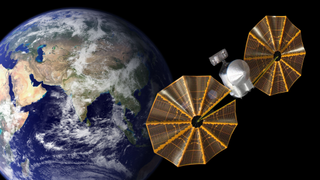In this detailed image of outer space, a black background sets the stage, highlighting the vibrant Earth visible in the lower left corner. The Earth's surface showcases the arid deserts of the Middle East, the greenish expanse of India and Asia, and is surrounded by the deep blues of various oceans, all partially hidden under swirls of white clouds. Dominating the right side of the image is a spacecraft or satellite. This object features a silver metallic, rectangular body with a prominent, circular dome at the front. Flanking this central structure are two large, coppery brown, round shapes, resembling spider-web-like propellers. The spacecraft appears to be subtly drifting through space away from Earth, which occupies the left half of the view.